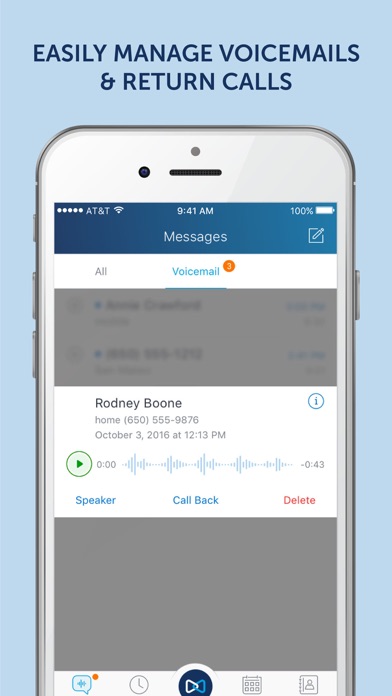The image features a promotional graphic for a voicemail management system, showcasing a light blue-to-dark blue gradient background. Prominently displayed at the top in dark blue capital letters is the message: "Easily manage voicemails and return calls."

Beneath this text is an image of a white and gray smartphone screen. The top section of the screen shows a dark blue header with the AT&T logo, Wi-Fi signal strength, the time "9:41 AM," the word "Messages," and a fully charged 100% battery icon.

The main interface of the phone screen is divided into several sections: 

- The first section is labeled "All Voicemail" in a white area with an orange circle.
- Below this is a gray box.
- Further down, a white box displays the name "Rodney Boone," accompanied by smaller, unreadable text due to blurriness.
  
Functional buttons are presented below Rodney Boone's name, including "Speaker," "Callback," and "Delete." Adjacent to these buttons are two circles, one with a "Play" icon and another with a lowercase "i" for information.

The bottom segment of the screen includes a gray area followed by a white area, containing five blurred buttons. Despite the lack of clarity, one button resembles a clock, another a text box, and the center button is dark blue with a white and light blue circular design.

The overall presentation aims to demonstrate the ease and functionality of managing voicemails and returning calls through a well-organized interface.